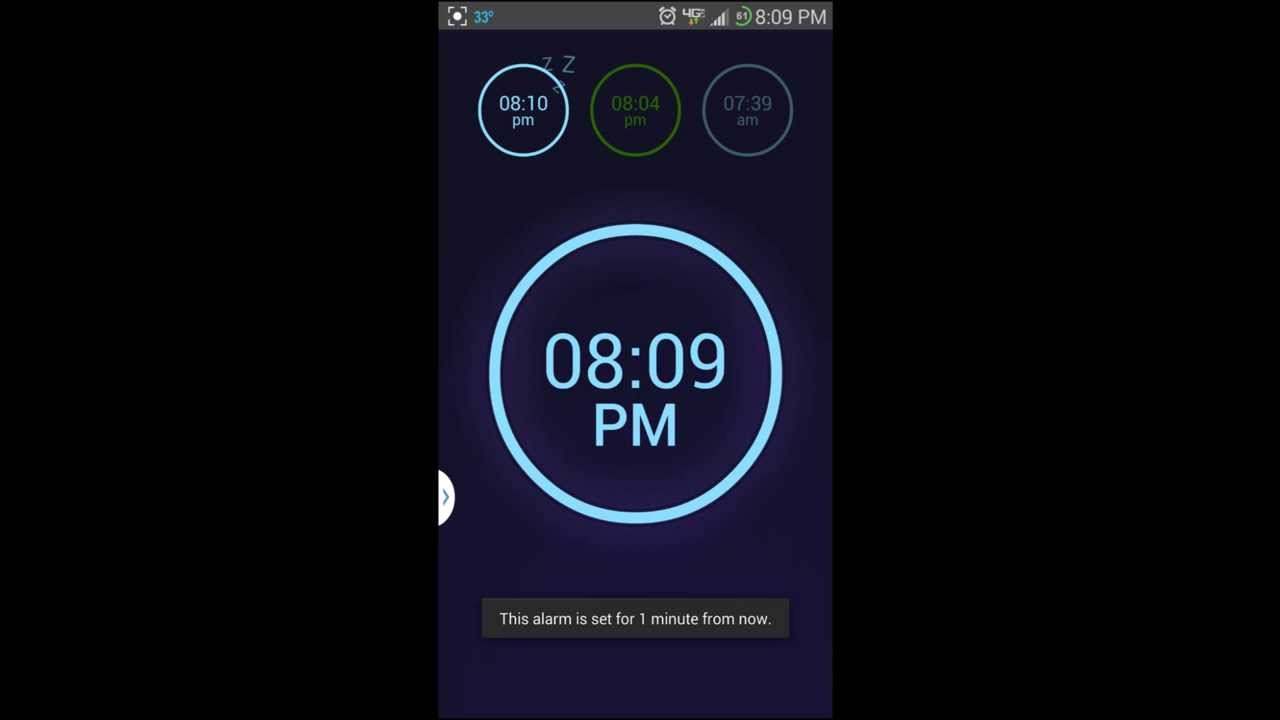This image is a screenshot of a mobile device displaying a dark navy blue background. The screenshot is bordered by black bars on both the left and right sides. At the top of the screen, there are three circles:

1. **Top Left Circle**: A sky blue circle showing "8:10 PM" with small "Z's" symbols floating around, indicating sleep or rest.
2. **Top Center Circle**: A green circle displaying the time "8:04 PM."
3. **Top Right Circle**: A grayish-blue circle showing "7:39 AM."

In the bottom center of the screen, there is a prominent, bright sky blue circle displaying "8:09 PM." Below this time, there is a caption that reads: "This alarm is set for one minute from now," indicating an active alarm due at 8:10 PM.